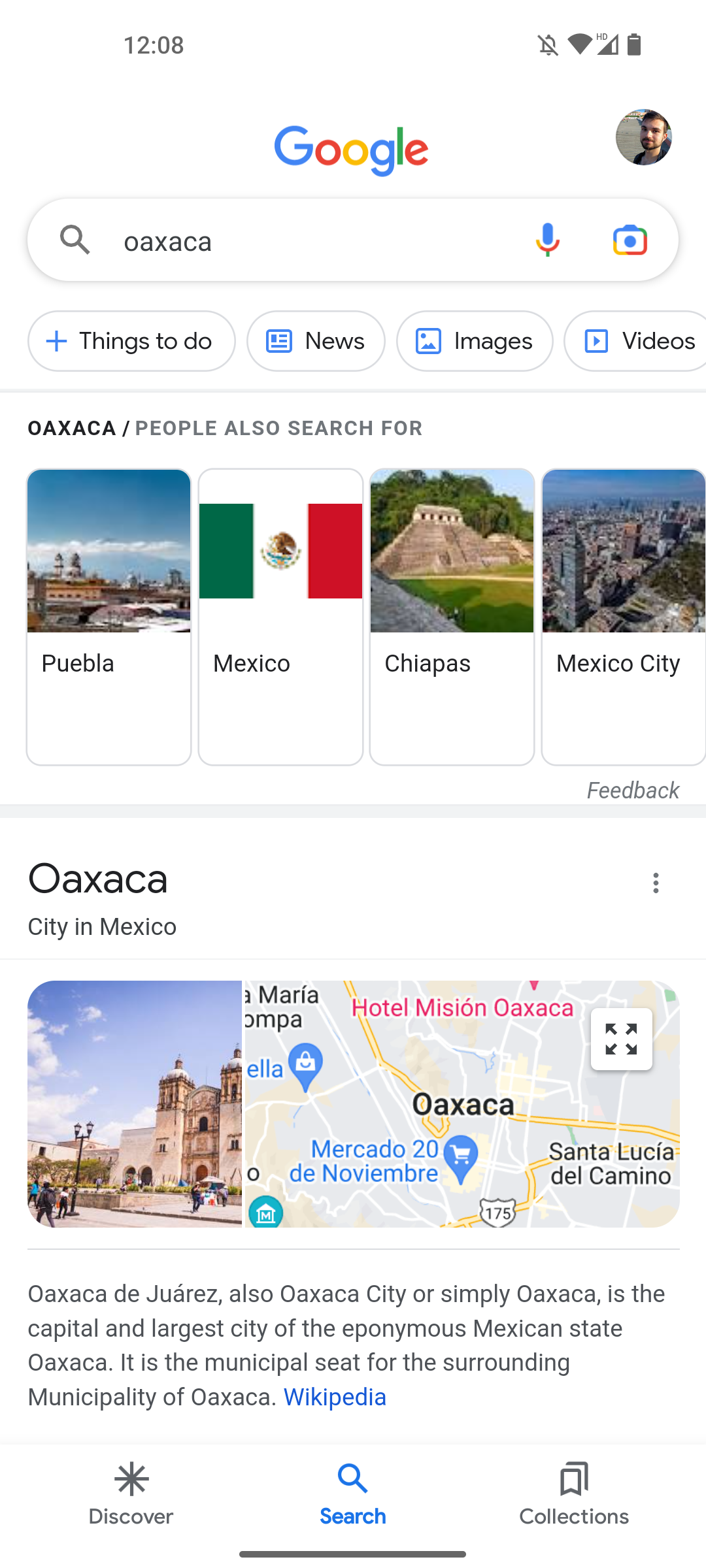The image depicts a smartphone screen with the following details:

In the top-left corner, the time is displayed as 12:08. On the top-right corner, various status icons are visible, including a notification bell (appearing to be turned off), Wi-Fi signal strength, cellular signal strength, and a battery indicator.

Below these details, there is a Google search bar with the query "OAXACA" entered. Beneath the search bar, search options are presented, such as "Things to do," "News," "Images," and "Video."

Further down, the screen shows a section titled "OAXACA / People also search for." This area lists four alternative locations: Puebla, Mexico; Chiapas; and Mexico City. Each location is accompanied by a small representative image, except for Mexico City, which features the Mexican flag as its image.

Below this section, there is an image of Oaxaca, identified as a city in Mexico. Next to the image, a map is visible, allowing for zooming in and out. Accompanying this is a brief piece of text from Wikipedia providing an overview of Oaxaca.